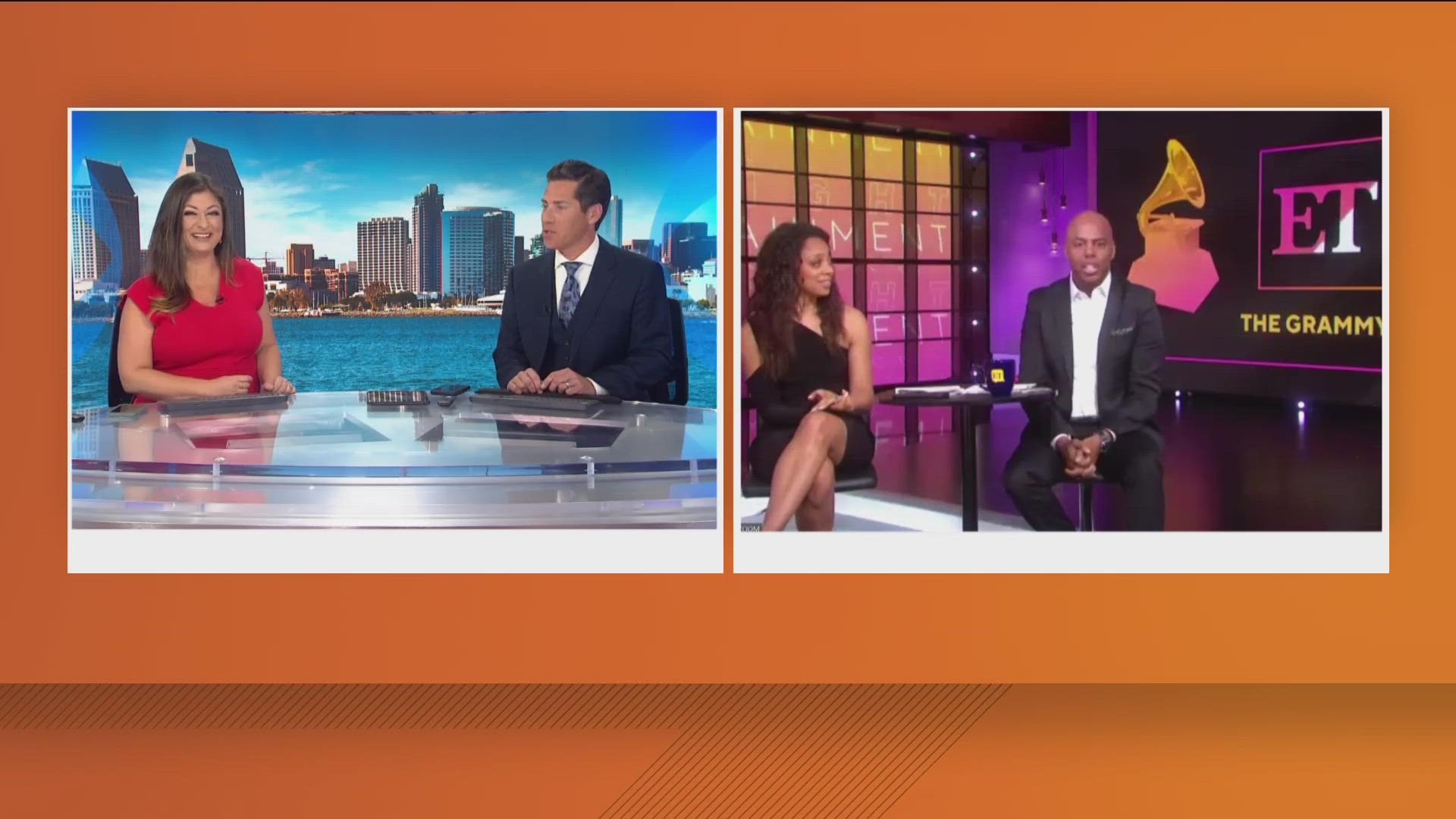The image consists of two side-by-side photographs on a horizontal rectangular orange background that transitions from darker on the left to lighter on the right. Below the photographs is a small rectangular border. 

On the left, a man and a woman are seated behind a shiny, clear glass desk. They appear to be hosting a news show, with a scenic backdrop featuring a cityscape of high-rise buildings and a large body of water. The woman, a Caucasian with long brown hair, is dressed in a red dress. The man, also Caucasian with short brown hair, is wearing a dark blue shirt complemented by a white-collared light blue tie.

On the right, another pair consisting of a black man and a black woman are seated around a small, high, round table, likely at an event related to the Grammys. Behind them, the wall displays a sign reading "E.T. The Grammys" in purple and yellow colors, indicating an Entertainment Tonight segment. The room has a purple hue. The man, bald and dressed in a tuxedo with a white shirt but no tie, is seated on a higher leather-backed chair. The woman wears a black dress that elegantly drapes over one shoulder, revealing the other, and has long curly brown hair.